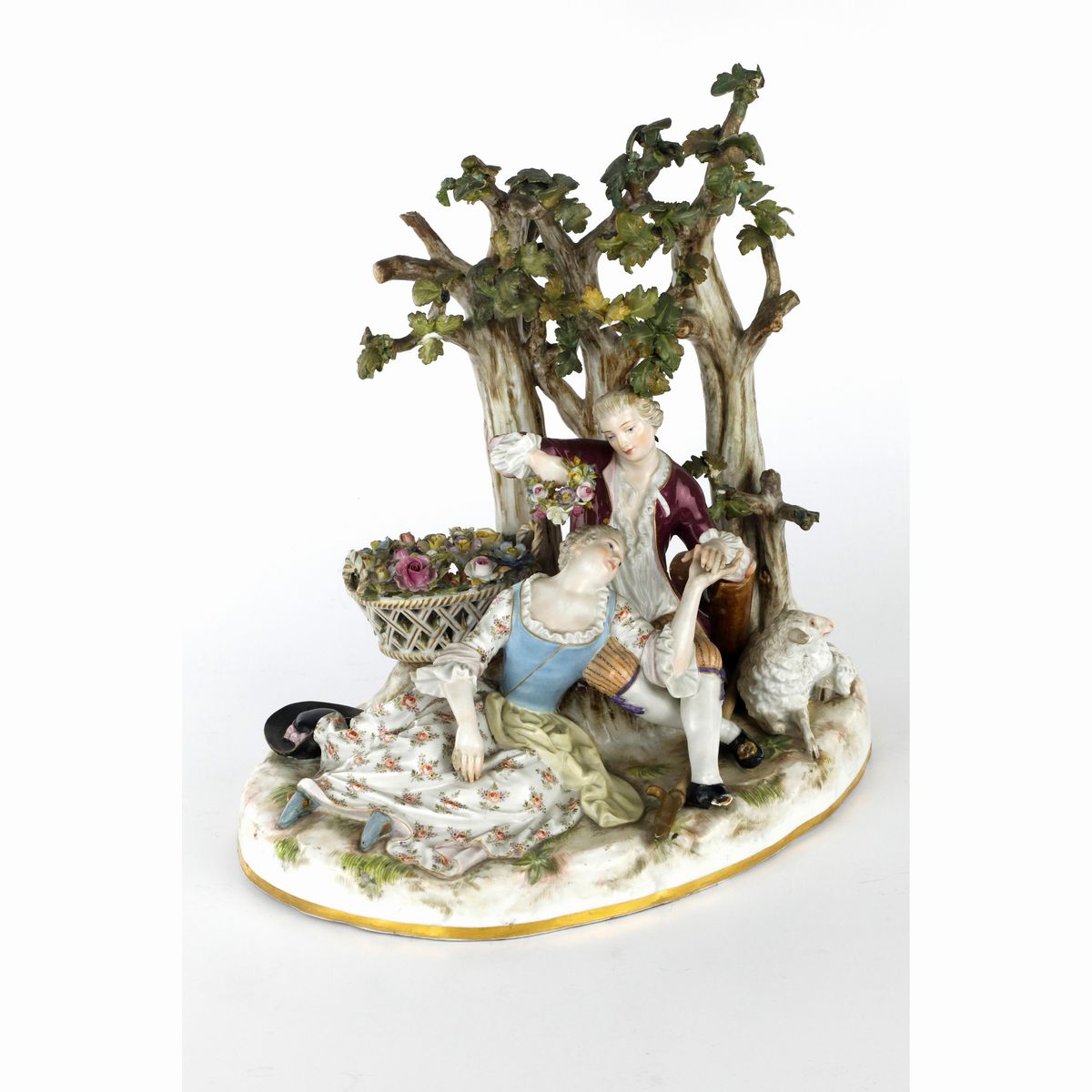This is a detailed color photograph of a finely crafted porcelain figurine, likely of an 18th-century romantic scene. The figurine rests on an ovular white base accented with a gold rim. It features a man and a woman positioned under three small trees with green leaves. The man, who is seated against the trees, is dressed in a burgundy colonial-style jacket over a frilly white shirt, beige capri pants, and black shoes. He holds a flower wreath above the woman's head while clasping her hand lovingly.

The woman, sprawled out on the ground in front of him, wears a white floral dress with flowy sleeves and a blue corset. Her head tilts back as she reaches up to touch the man's hand. A woven basket filled with flowers sits to their left, near a black hat with a pink bow, possibly belonging to either the man or the woman. A white sheep lies contentedly on the ground near the couple, to their right, adding a pastoral charm to the scene. The figurine's intricate details and glossy glaze suggest an antique, decorative piece, likely designed to adorn a living space such as a dining room table or a bookcase.